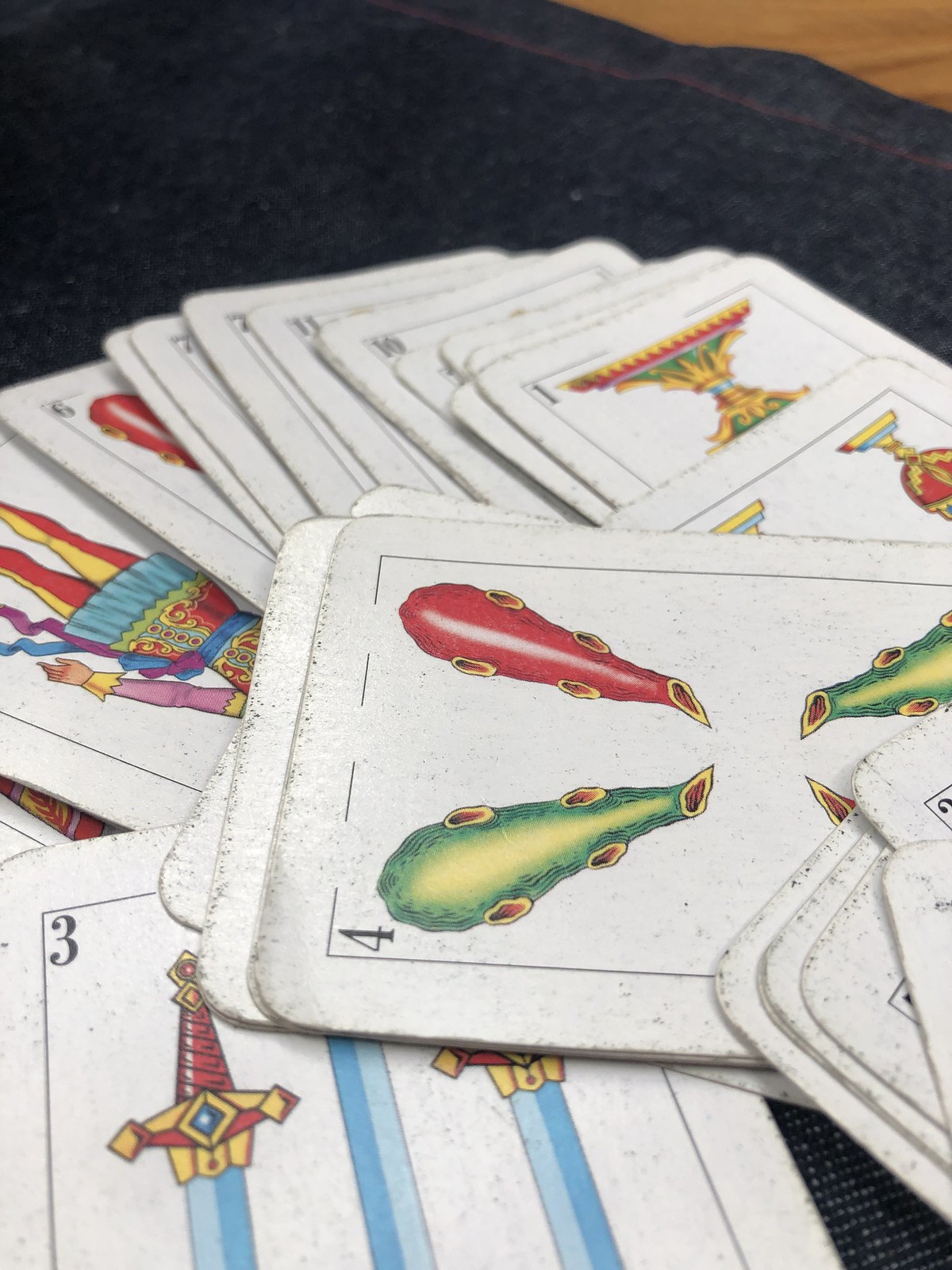The image captures a top-down view of a pile of approximately 20 cards laid out on a black cloth. In the top upper right-hand corner, a portion of a brown table is visible. Dominating the center of the photograph, the cards, some stacked and some splayed, reveal their illustrated fronts and edges.

In the bottom left of the image, a white card prominently features a sword with a brown handle, a blue gem, and a silver blade, marked with the number "3" in the upper corner. Adjacent to this sword card, there is another card depicting a similar weapon.

Towards the middle right, a card turned on its side displays the number "4" and features a green object, resembling a perforated baseball bat, with an open end. Nearby, another card showcases a similar object in red, sporting a similar design of holes and an open bottom.

In the foreground of this red card, partial legs clothed in what appear to be tights and a blue dress can be seen, hinting at the presence of a human figure within the card illustration. The collection of cards, each teeming with various details, creates an intriguing and visually rich tableau.